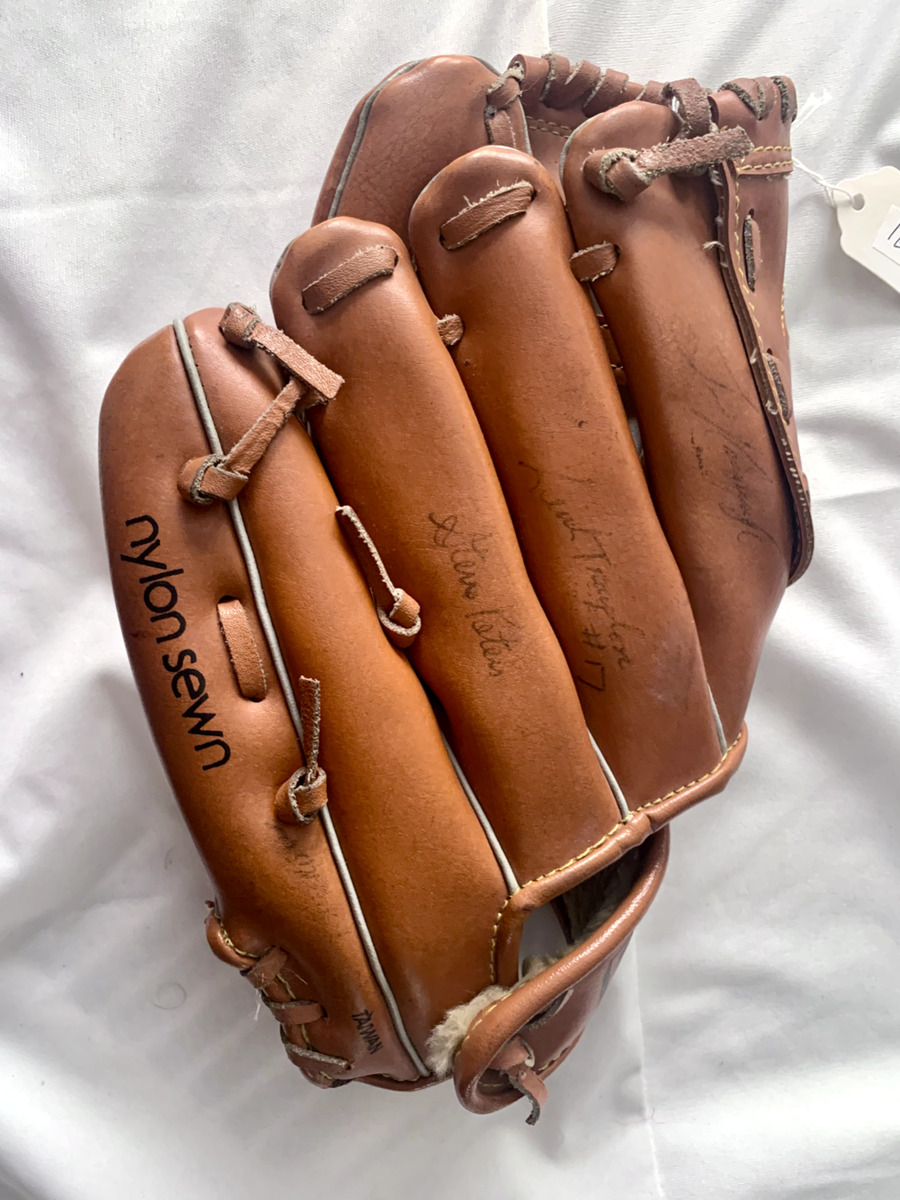This detailed close-up image captures a light brown, slightly worn baseball glove set against a white cloth background, resembling a bed sheet. Prominently featured on the glove is the text "nylon sewn," indicating its stitching material. Notably, the glove boasts several signatures on the outer finger areas, suggesting it has been autographed by players, adding a collectible value. At the top of the glove, a white price tag, attached with a thin white string, is visible but partially cut off, hinting that the glove is likely for sale. The glove's interior is lined with tan fleece, providing comfort for the hand. The overall presentation in the image seems to aim at showcasing the glove, possibly for an online listing.